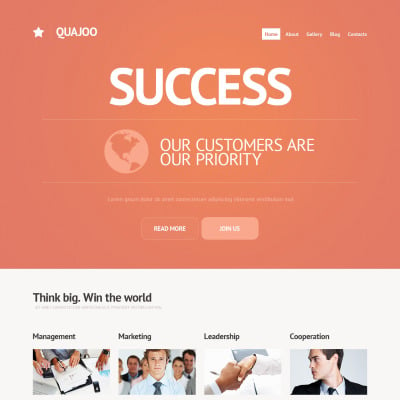This screenshot captures a cropped section of a web page, potentially representing either a live website or a graphical layout of a web design. Notably absent are typical web browser elements such as navigation bars and scroll buttons, which leaves the status of the web page—whether interactive or static—ambiguous.

The header of the web page features a minimalistic design comprising a white star logo accompanied by the text "Kwa Jo." Positioned on the top right is a navigational menu with the options: Home, About, Gallery, Blog, and Contacts.

Dominating the upper portion of the screenshot, there's a prominent box with an orange background. In this section, the word "SUCCESS" is boldly displayed in large, white capital letters. Accompanying this, a tagline reads, "Our customers are our priority." Beneath this tagline, users are prompted to engage with options like "Read More" or "Join Us," accessible via distinct buttons.

The cropped lower section of the screenshot lays against a white background and includes another motivational tagline: "Think big, win the world." Below this, there are four delineated boxes titled "Management," "Marketing," "Leadership," and "Corporation." Each box is illustrated with corporate graphics that depict people in workplace scenarios, adding a visual element to the content.

Overall, the captured section offers a glimpse into a professionally designed web page that emphasizes success and customer value, illustrated with rich visual elements and clear navigation options.